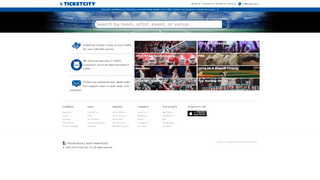The image depicts a somewhat blurry ticketing website, identifiable by the prominent blue-colored "Ticket City" banner at the very top. The banner features a central search bar, facilitating user navigation. Below the banner is a large image, presumably of a stadium, although its clarity is not sufficient for a definitive identification. Further down the page, eight smaller photos are arranged towards the right-hand side, each representing various events available for purchase. On the left-hand side, there are three blue icons accompanied by brief two-to-three-line paragraphs that likely describe the website's offerings and features. The overall background of the website is white, creating a clean and cohesive appearance that highlights the blue icons and symbols, matching the top banner's color scheme.